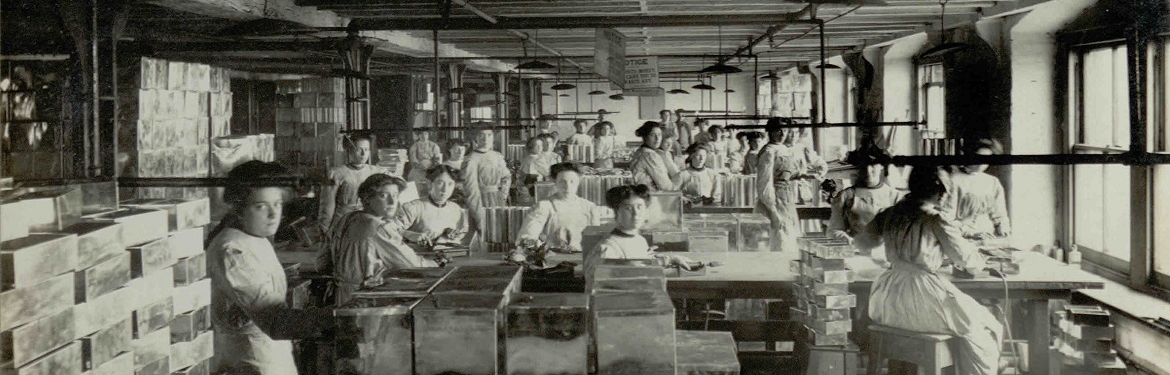The black and white panoramic photograph depicts a historical factory setting, with an unclear time period. The image primarily features female workers, dressed in long white dresses with high necks and long sleeves, sitting around long tables. The tables are surrounded by open boxes, possibly bins, and the foreground and background are filled with these tables and workers. Overhead, black lights hang but do not appear to be on. The room is lit by natural light streaming through windows on the right side. Piping and probably overhead nozzles for dispersing liquid, likely for fire suppression, run along the ceiling. Though the specific task the women are engaged in remains ambiguous, the scene conveys a sense of organized labor within a clean and structured indoor environment.